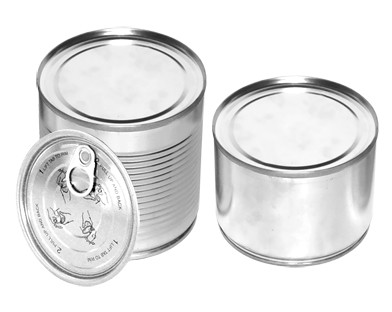This image depicts two silver tin cans positioned upright on a plain surface, viewed from an angle that showcases the top edges. The can on the left is taller and features a ribbed center with horizontal lines encircling its body, adding texture to its otherwise smooth metallic surface. The taller can has an accompanying pull-tab lid, which rests on its side, leaning against the can's body and displaying some black text detailing instructions, though the can itself remains sealed. The can on the right is notably shorter, seamless and devoid of any ridgings or additional details. A soft light illuminates the scene, casting a gentle glare on the metallic tops of both cans. This image appears to serve as a templated marketing material, highlighting the basic yet functional design of the tin cans.